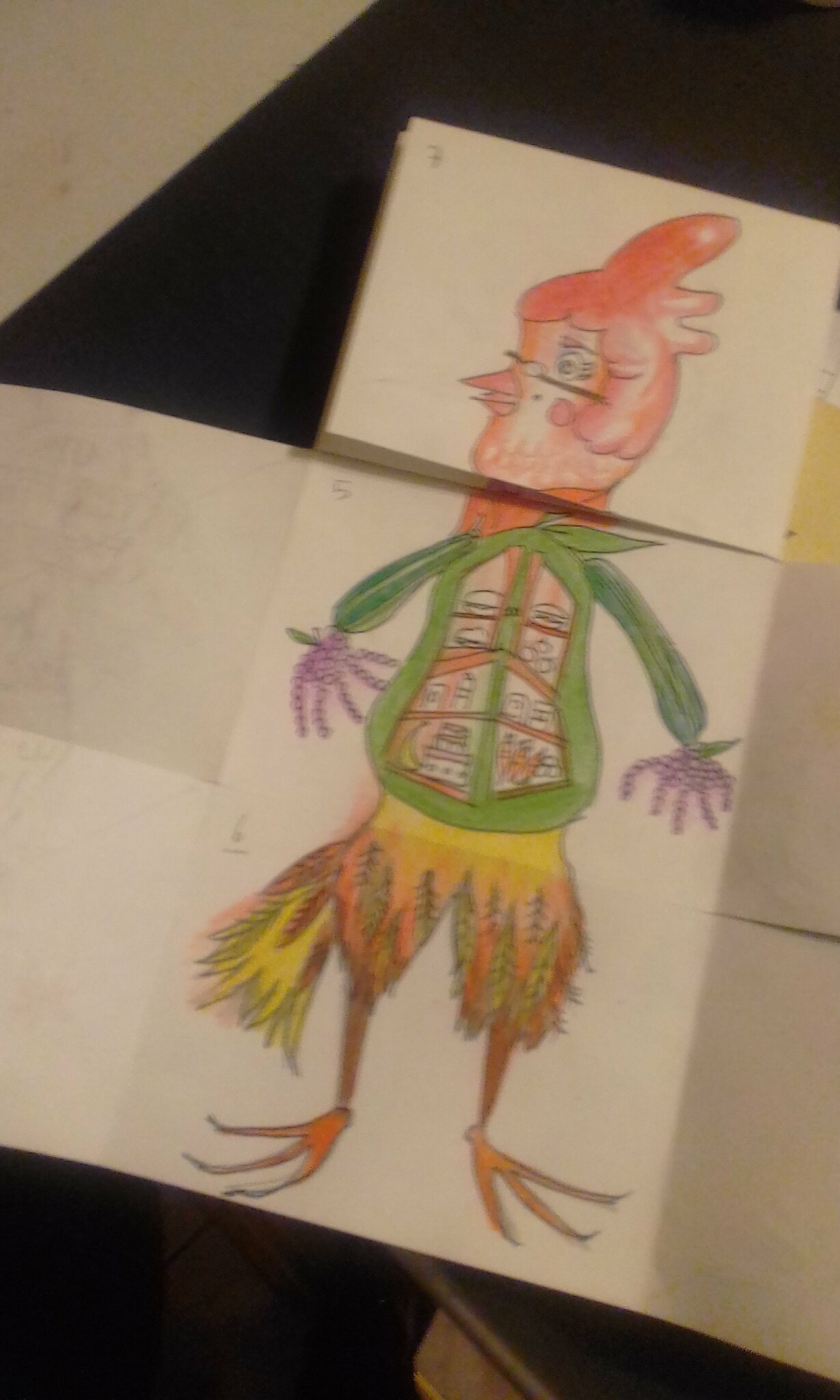This image features a whimsical, hand-drawn flipbook illustration that appears to combine three distinct segments: a head, a body, and legs, each depicted on separate small pads of paper. The concept allows for the mixing and matching of different parts to create unique characters. In this particular arrangement, the head is depicted in vibrant red, resembling a chicken adorned with glasses. The green body is creatively composed of various food items, including grapes for hands and cucumbers for arms, with windows revealing an assortment of other foods inside. Completing the figure, the legs are rendered in yellow and orange, akin to chicken legs. The image is purely visual with no accompanying text.